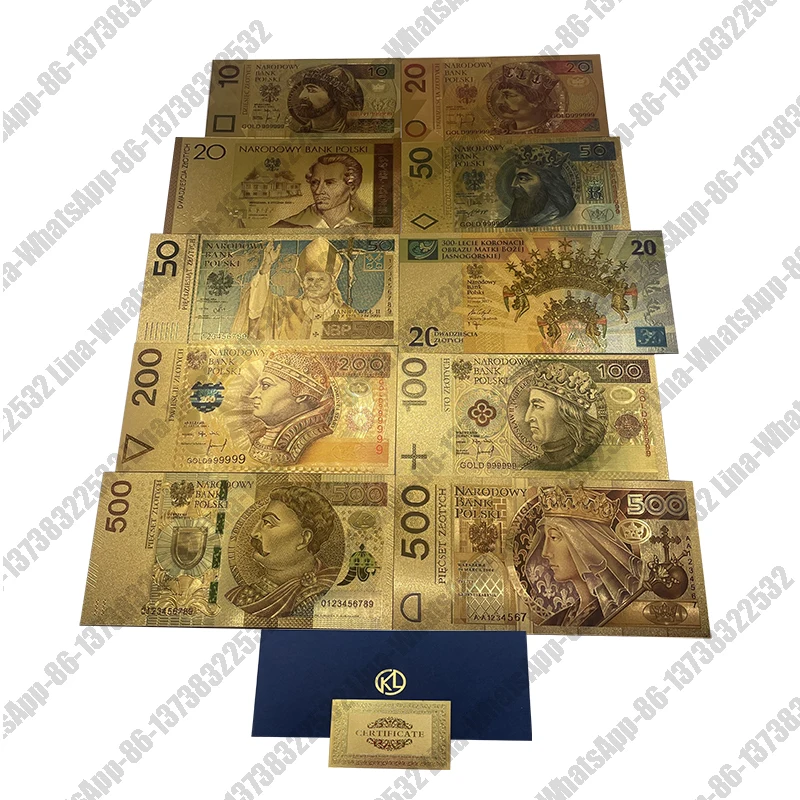The image depicts an array of paper currency organized in two columns with five rows each, displayed against a white background with a light gray watermark repeating diagonally that reads "WhatsApp 86 1 3 7 3 8 3 2 2 5 3 2" alongside the name "Lena." The currencies are vibrant and diverse, each featuring distinct portraits and designs, possibly of Polish origin, as suggested by the label "Bank Polski" on one of the notes. 

In the left column, the topmost bill is a "10" denomination, featuring a portrait of a man. Below it is a "20" bill with the profile of another man. The third bill down is a "50," showcasing a figure that resembles a pope or religious leader. Beneath it is a "200" currency, adorned with a man wearing a round crown with a blue shield. The bottom of this column displays a "500" denomination, with a man sporting a mustache.

In the right column, the topmost bill is another "20" currency, featuring a crowned man. Below it is another "50" bill with a different crowned figure. The third bill is yet another "20," distinguished by two crowns, one atop the other. Next comes a "100" bill, showcasing a crowned profile, possibly a king. The bottom right features another "500" currency, this time depicting a crowned queen with a ball and cross symbol.

Below the array of bills, there’s a blue rectangle with a small yellow symbol, alongside a yellowish-brown rectangle radiating from a smaller orangish rectangle, marked with upper and lower symbols, suggesting some form of artwork or certification.